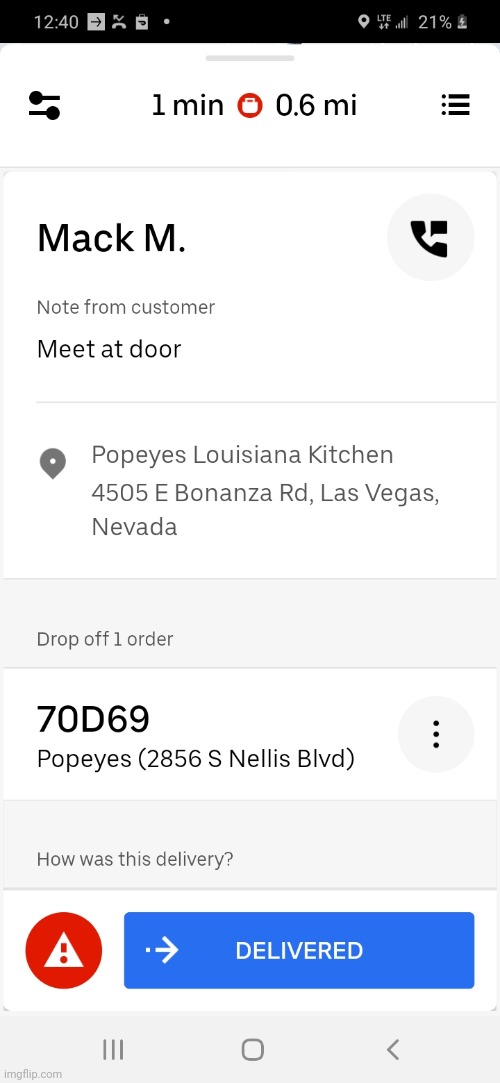This is a detailed screenshot from a gig worker app displayed on a cell phone. The status bar at the top features a black horizontal bar with white icons: the time (12:40), a square with a right-facing arrow, a phone receiver, a square containing a curved triangle, a white dot indicator, and a speech bubble with a white dot resembling a pin. Next to these icons is the LTE signal indicator, Wi-Fi signal bars, and a battery indicator showing 21% with a white downward arrow.

Below this, the interface features a white background divided by grey lines. On the left side, there's a settings icon. In the center, bold black text reads "1 minute" next to a red circle containing a white shopping bag. To the right, it displays "0.6 miles," and further to the right are three horizontal lines, each accompanied by a bullet point.

Underneath, there's a grey outlined area with bold text stating "MAC-M," alongside a phone receiver and a grey speech bubble. Below this, in grey text, is a note from the customer, "meet at door." The pickup location is identified as Popeye's Louisiana Kitchen, including its Nevada address, marked by a grey pin icon with a white dot.

Following this is a horizontal grey bar reading "Drop off one order" in black text. Under this is another white horizontal section with the bold black letters "70D69," the name "Popeye's," and the address repeated. To the right, there is a grey bubble containing three vertical dots.

The next section features a grey line with the prompt "How is this delivery?" At the bottom of the interface, a red circle on the left contains a white triangle with a red exclamation point, while a dark blue rectangle to the right highlights a white right arrow and the word "Delivered" in white.